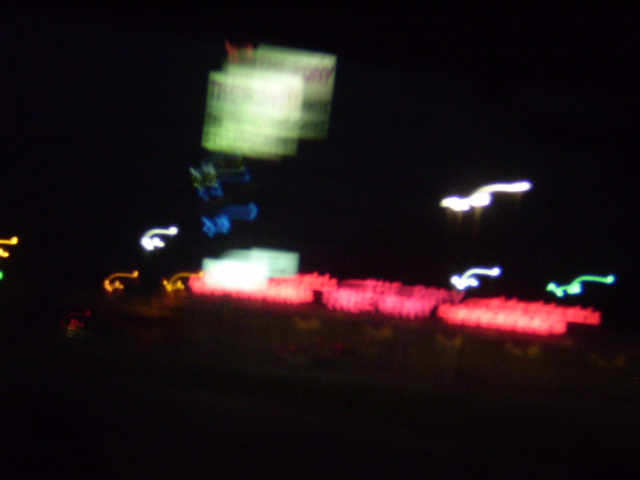This image is quite challenging to see clearly due to its overall darkness. It appears to mimic an etch-a-sketch drawing, featuring what seems to be a boat. The scene contains sporadic blue elements that resemble life forms. In the background, several objects look like seagulls in flight, depicted in varying colors including green, white, blue, and orange. Above the boat, there are two signs, although the red lettering on them is entirely blurred and illegible. Below pink lights, there's a form that likely represents a boat, but it remains difficult to discern due to the profound darkness enveloping the image.